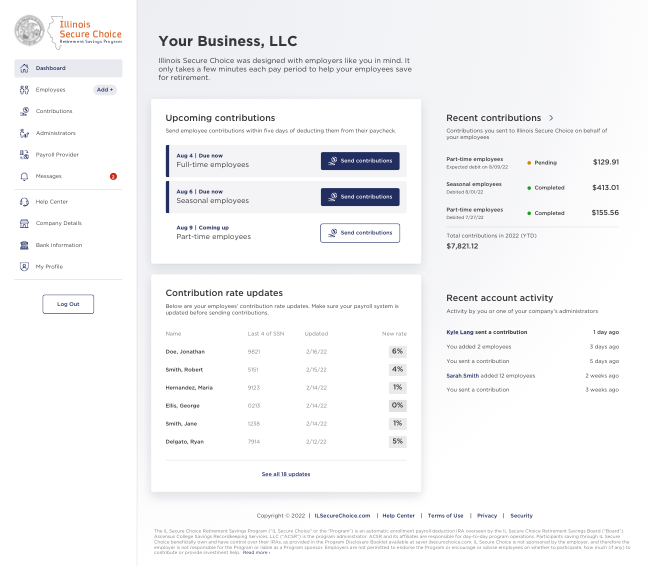The image features an interface with a predominantly white background on the left side, occupying a small section. At the top of the artwork, the text "Illinois Secure Choice" is prominently displayed. Below this header, there is a blurred section with illegible text that appears to be three words long and in black. Following this is the word "Dashboard" in navy blue, enclosed within a gray box. The interface then lists several menu items in black: "Employees," "Contributions," "Administrators," "Payroll Provider," and "Messages." There is a red notification circle indicating an unread count of either two or three.

Further down, additional menu options in black include: "Help Center," "Company Details," "Bank Information," and "My Profile." At the bottom of this section, there is a white box outlined in navy blue, with the word "Logout" written in navy blue.

The right side of the background is gray and features the text "Your Business LLC" in black. Below this, it states, "Illinois Secure Choice was designed with employees like you in mind. It only takes a few minutes each pay period to help your employees for retirement." The section titled "Upcoming Contributions" reminds users to send employee contributions within five days of withholding them from paychecks. 

A slightly blurred section lists employee types: "Full-time employees," "Seasonal employees," and "Part-time employees." Following this is the section "Contribution Rate Updates," informing users to update their payroll systems. The displayed contribution rates include 6%, 4%, 1%, 0%, 1%, and 5%.

The last visible section "Recent Contributions" lists monetary amounts for different employee categories: part-time contributions of $100.29 and $129.91, seasonal contributions at $413.01, and part-time contributions of $185.56.